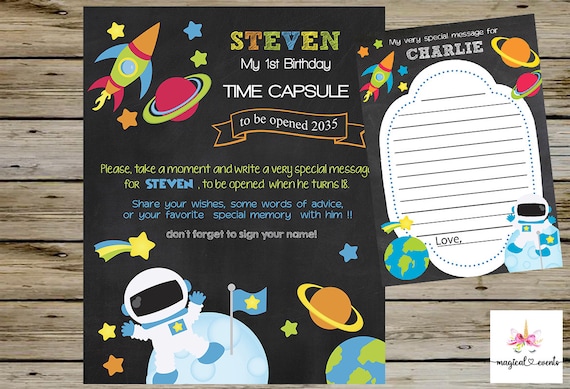The image shows a beautifully illustrated birthday invitation set on a rustic wooden table made of seven horizontally arranged dull brown planks. The centerpiece is a black poster with a whimsical space theme, celebrating Stephen's first birthday. The poster reads: "Stephen, my first birthday, time capsule to be opened in 2035." It invites guests to "please take a moment and write a very special message for Stephen to be opened when he turns 18," encouraging them to share wishes, advice, and favorite memories, and to sign their names.

The poster is adorned with colorful cartoon space figures, including a rocket ship, a planet with rings reminiscent of Saturn, an astronaut standing on the Moon with a flag, a shooting star, and Earth in the background. Next to this is a smaller piece of paper titled "My very special message for Charlie," which also follows the space theme. It features similar decorations: a rocket ship, Saturn, an astronaut on the Moon, and a shooting star, enclosing a text box for handwritten messages, concluded with the word "Love," allowing space for the writer’s name. Both items lie on the wooden surface, ready for guests to leave their heartfelt messages.